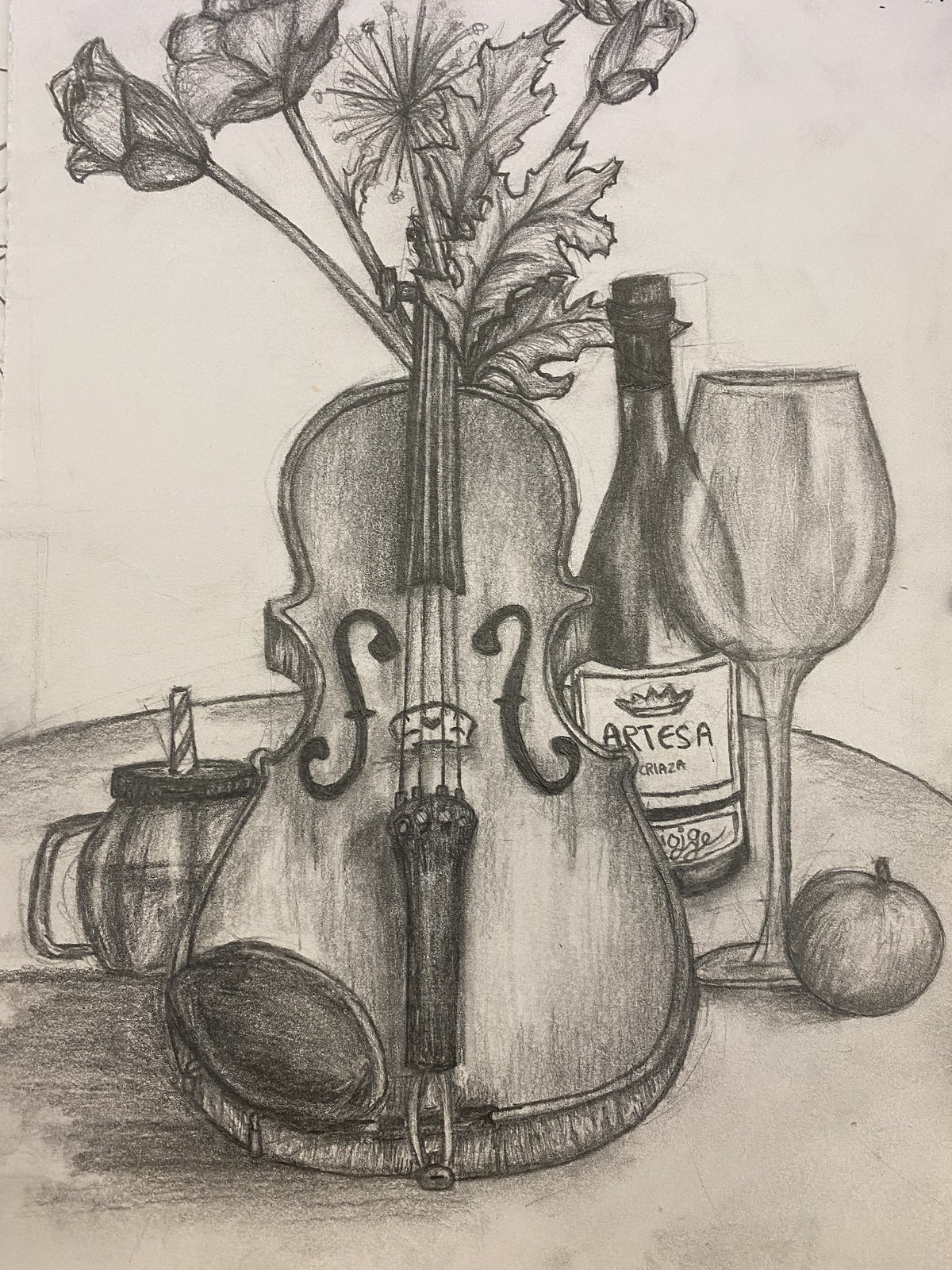This charcoal pencil drawing, rendered on off-white textured paper with subtle smudging, captures a rich still life scene. Central to the composition is a round table outlined with bold line work and light shading, providing a sense of depth. To the right of the table rests an apple, adjacent to a finely detailed wine glass. Behind the glass stands a wine bottle labeled "Arteza Criazza" and adorned with a crown logo. A mason jar-style cup, complete with a lid and striped straw, adds a touch of rustic charm. Dominating the center of the image is a violin, its distinctive S-shaped sound holes and strings expertly depicted. The violin's handle gracefully fades into a tangle of foliage and flowers at the upper part of the drawing, seamlessly blending natural elements with musical artistry.